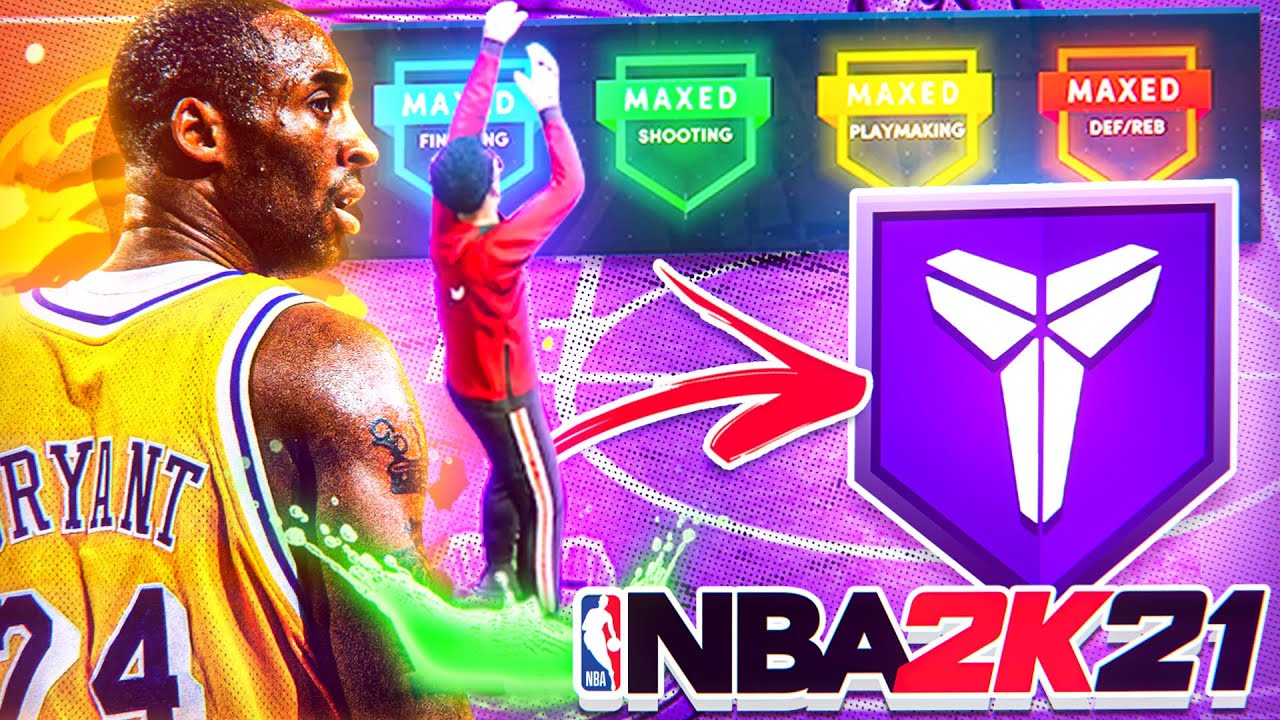In this vibrant and detailed screenshot, we are immersed in a dynamic video game scene from NBA 2K21. The top left of the image is dominated by a colorful, digitalized background featuring a blend of orange, yellow, and white hues. The focal point of the scene is basketball legend Kobe Bryant, positioned on the left side of the screen with his back to the viewer. Kobe is glancing towards the right, with his head turned slightly east.

He is depicted wearing a yellow jersey adorned with blue and white borders, and part of his last name, "BRYANT," is visible. Kobe, an African-American man, has a notably sweaty head and hair shaved very short. A distinct tattoo embellishes his upper right shoulder, adding to the lifelike portrayal.

In the lower right corner of the screen, bold and three-dimensional text displays "NBA 2K21" in striking red, against a sleek black box background. Adjacent to these letters, the iconic NBA logo, featuring its classic red, white, and blue colors, is prominently positioned. This scene captures the essence of both the legendary player's persona and the immersive graphics of the video game.